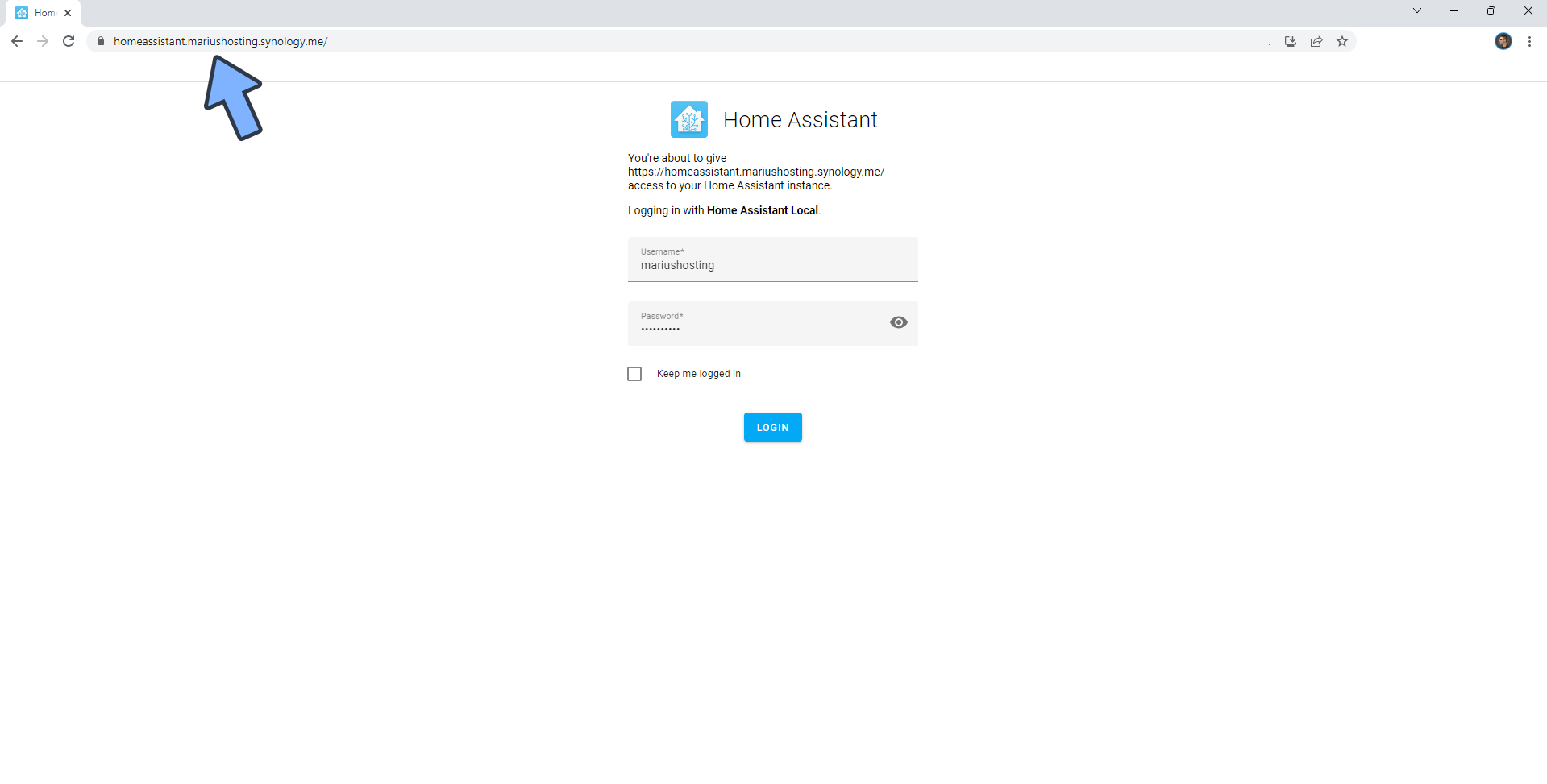The image captures a web browser displaying a single open tab with the address "homeassistant.marcushosting.synology.me." The browser's navigation bar includes a back button (leftward arrow), forward button (rightward arrow), reload button (circular arrow), favorites button (star), close button (X), and minimize button (underscore).

The webpage, titled "Home Assistant," features a blue logo depicting a white house. The main content of the page indicates that the user is about to grant the site "https://homeassistant.marcushosting.synology.me" access to their Home Assistant instance. The login section displays a message to log in with Home Assistant's local credentials. There is a username text box populated with the name "Marcus Amarius Hosting" and a password text box showing a series of asterisks for security. Additionally, there's an option labeled "Keep me logged in" (currently unchecked) and a prominent blue "Login" button.